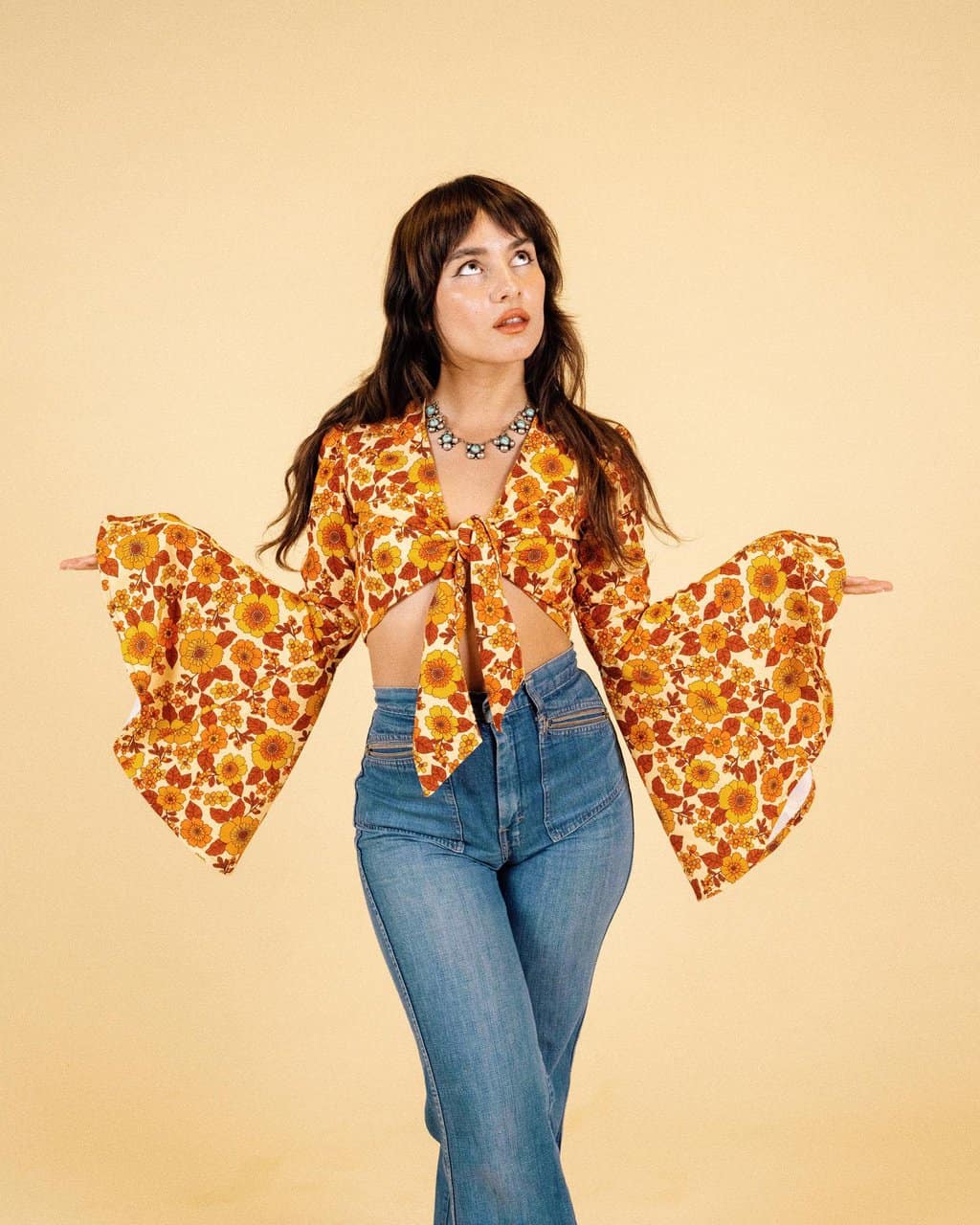The image features a young woman in her 20s standing at the center with her arms outstretched to her sides, looking up towards the sky with an expression of irritation, as if asking, "why?". She is dressed in a vibrant, floral-patterned halter top with colors of orange, yellow, and white, reminiscent of 60s and 70s fashion. The top is tied at the front, leaving her midriff exposed, and it has long, billowy sleeves that flow down her arms. She pairs the top with bright blue, high-waisted jeans that are likely bell-bottoms, featuring front pockets that may have zippers. Her jewelry includes a striking blue necklace with square jewels encircling her neck. Her hair is styled with short layers and bangs in the front, extending into long layers past her shoulders in the back. She wears red lipstick, adding a pop of color to her overall look. The backdrop of the image is a blend of whitish-orange hues, giving the setting a professional studio vibe.